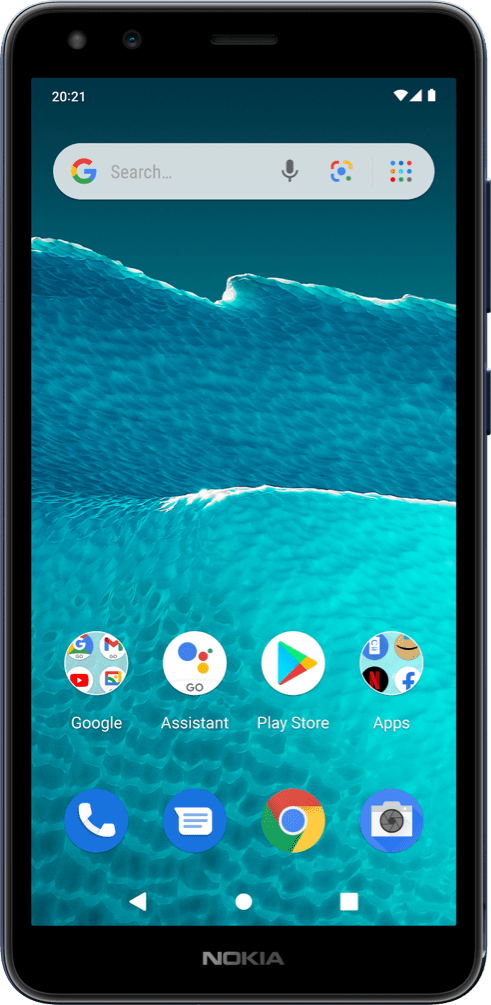Here, we have a detailed photograph of a smartphone, resembling an iPhone but branded with Nokia. The device features a standard rectangular shape with a black outline. At the very bottom of the phone, there's a black bar displaying the Nokia logo in a classic silvery font. 

The screen's background showcases a picturesque scene of ocean waves rolling onto a beach, with a mesmerizing blend of turquoise hues. 

At the top of the screen, the time is marked as "2021." The top right corner includes standard indicators: a Wi-Fi symbol, signal bars for 4G or 5G, and a fully charged battery icon.

Directly below these icons, there's a gray search bar. On the left side of the bar, the Google logo is colored in Google’s signature palette, followed by the prompt "Search..." There is also a microphone icon and another Google icon, which could be for voice assistant functions. Towards the right end of the gray bar is a small grid icon representing Google apps.

Near the bottom of the screen, several application logos are displayed in neat rows. The first label reads "Google," with associated Google app icons displayed above it. Then, there is the label "Assistant," accompanied by the Google Assistant logo. Following that is "Play Store," paired with the Play Store logo. Down below, a label that reads "Apps" showcases a variety of application icons, including popular ones like Netflix, Facebook, and Amazon Shopping.

In the next row, there is a blue circle featuring a white phone handset icon, indicating the phone application, among other application icons.